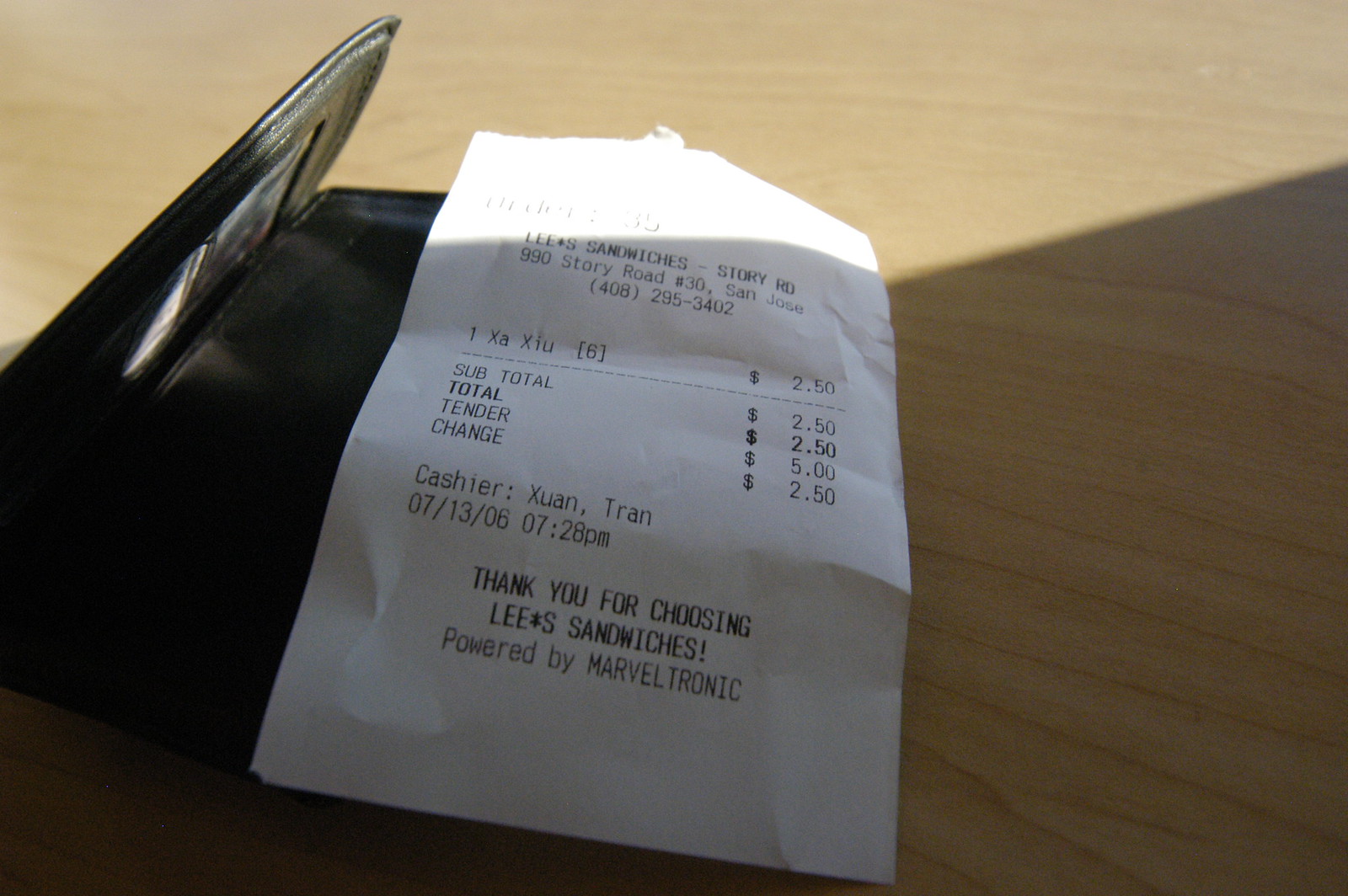The image features a receipt resting atop a wallet, both placed on a brown wooden table. The bottom of the receipt displays a message in bold black letters: "Thank you for choosing Lee's Sandwiches, powered by Marvel Tronic." The cashier’s name is printed above this line. The receipt also shows a transaction date of July 13, 2006, with a timestamp of 7:28 PM. It details a purchase of a sandwich priced at $2.50. The customer tendered $5.00 in cash and received $2.50 in change.